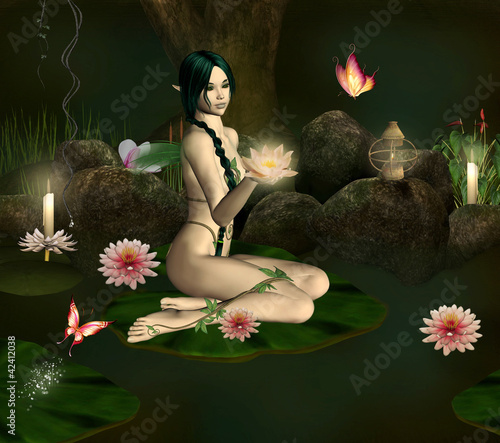The image is a detailed 3D rendering of a female character, most likely from a game or a 3D program. In the lower left corner, there's white text reading "Adobe Stock number 42412038." The central focus is a pale-skinned woman with long, dark forest green hair braided into a ponytail that drapes over her shoulder and chest. She has pointed ears, giving her an elfin or fairy-like appearance, and intricate green leaf motifs adorn her thin bikini.

The woman is seated on a large green lily pad in a body of water, with her legs folded underneath her. In her right hand, she holds a glowing lotus flower that radiates purple and white light. The background is predominantly dark, suggesting a night-time setting, and behind her appears to be a forest.

Additional details include various flora surrounding the scene: a pink flower to her right, another pink flower directly behind her, and yet another in front of her shin. There's also a white flower with a candle in it located in the upper left corner. A pink butterfly is visible in the lower left corner, adding to the mystical ambiance. There are also other lily pads visible on the water and some stones in the scene, with a lantern and a separate candle resting on some of them. A feathery wisp of light green color hovers behind her, further enhancing her fairy-like essence.